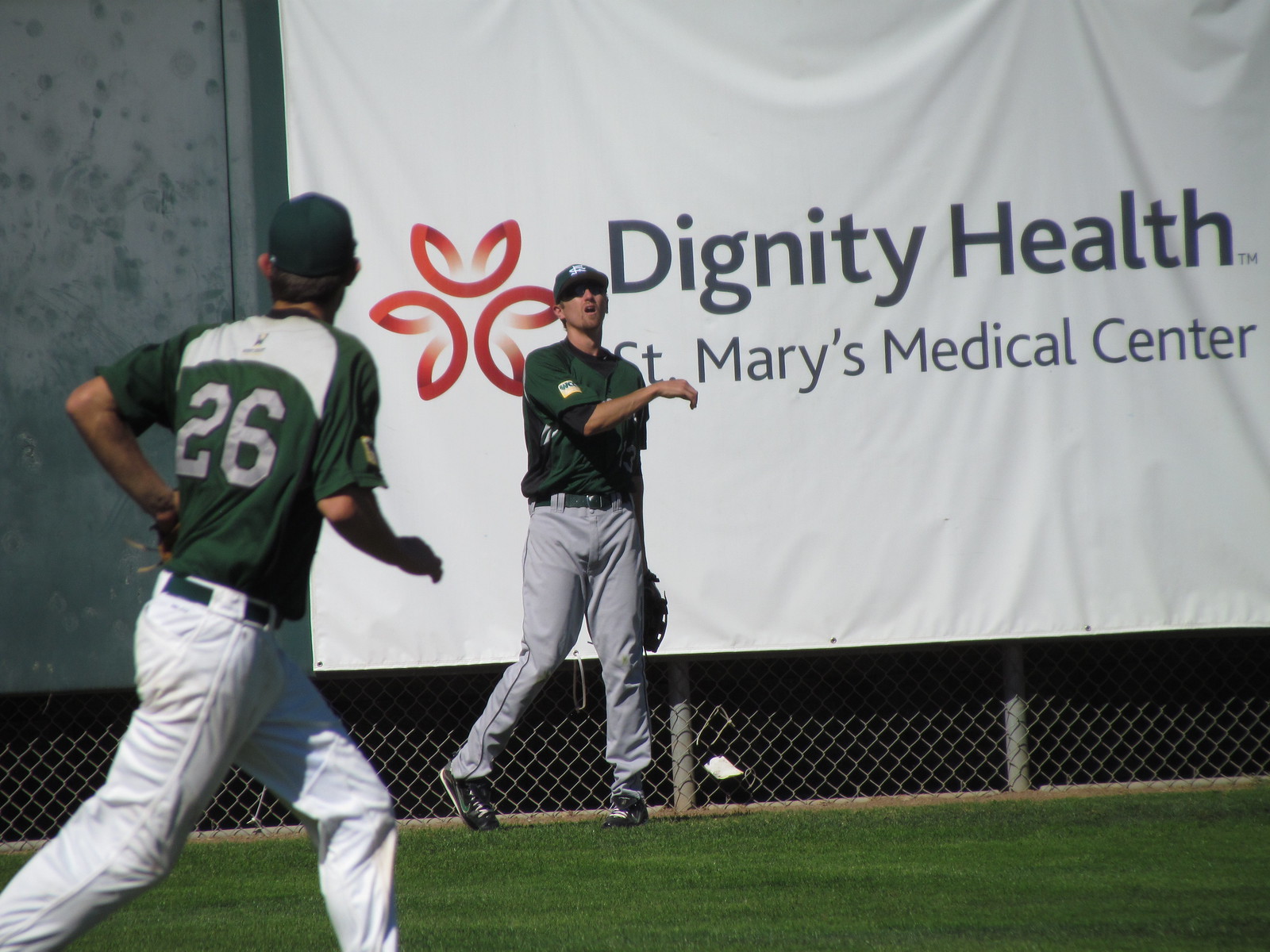In this image, we see a lively baseball game featuring two players on a meticulously maintained, vibrant green baseball field. To the left, a player in a deep green jersey marked with a prominent gray number 26 and a white stripe on top is sprinting to the right, looking backward. He is dressed in white pants and wears a dark blue baseball cap, with just the tip of his ears visible. In the background, another player, similarly attired in a matching dark green shirt and cap with a white insignia, stands poised with his glove held down behind his leg and his other arm raised across his chest, as if he has just completed a throw. He is sporting gray shorts and black shoes. Stretching along the chain-link fence behind them, a large white banner reads "Dignity Health St. Mary's Medical Center," with a distinctive red sunburst emblem on the left. This photograph captures a dynamic moment within the game, with both players centrally positioned against the backdrop of the lush field and the prominent advertisement.